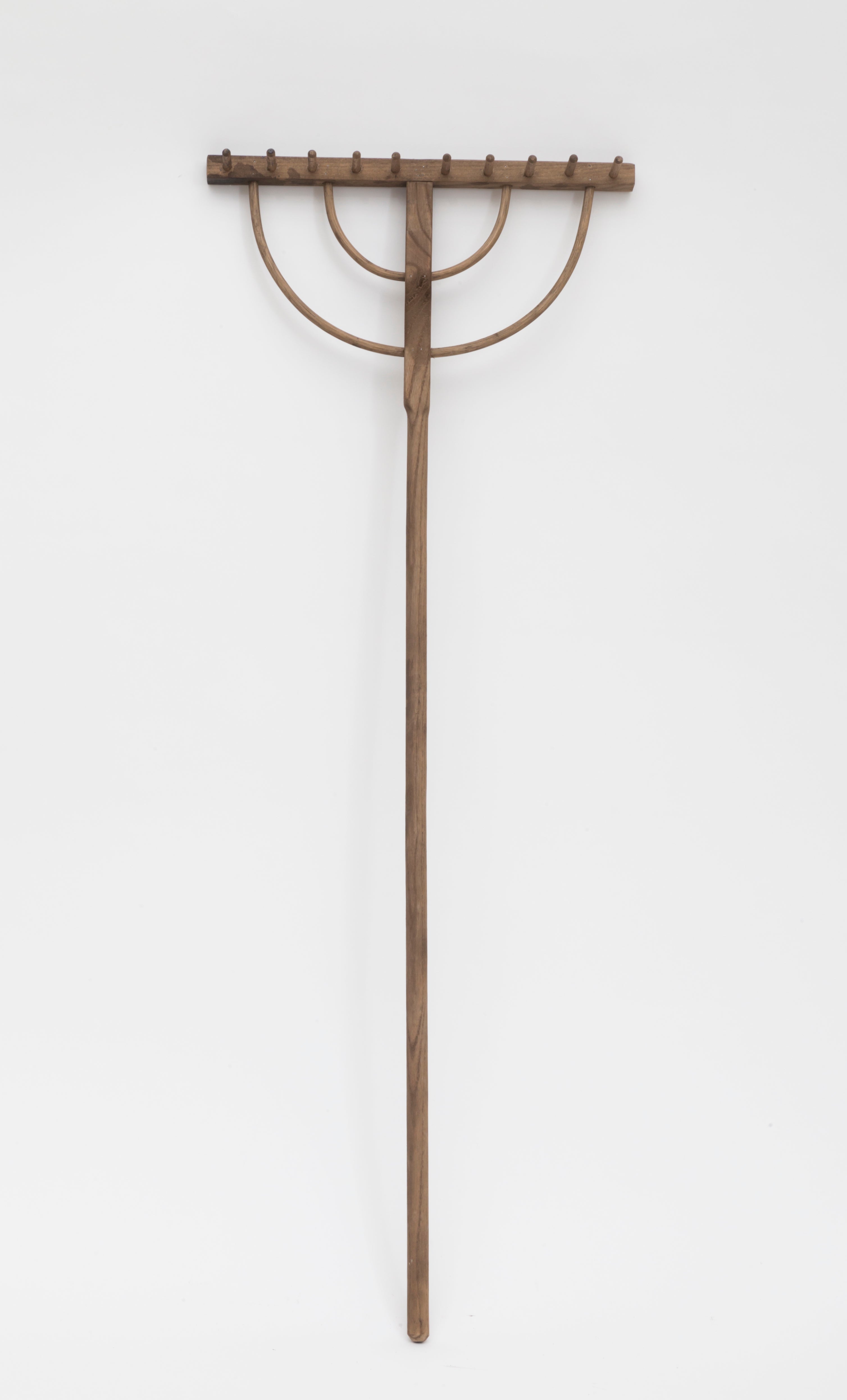The image depicts an antique, handmade wooden rake, set against a plain white background. The rake features a long, tubular wooden handle that slightly widens and flattens towards the top where it forms a T-shape with a horizontal crossbar. This crossbar, also wooden, has ten evenly spaced, whittled pegs protruding downward, creating the teeth of the rake. Below this crossbar, two arched wooden dowels on each side connect it to the handle, forming half-circle shapes that add to the rake's structural integrity. The entire object, bathed in a soft shadow, showcases a rustic aesthetic reminiscent of a bygone era when such tools were commonly used for raking ground or leaves. The distinct design and craftsmanship evoke a sense of history and functional beauty, captured in what appears to be a highly detailed, possibly photorealistic setting.